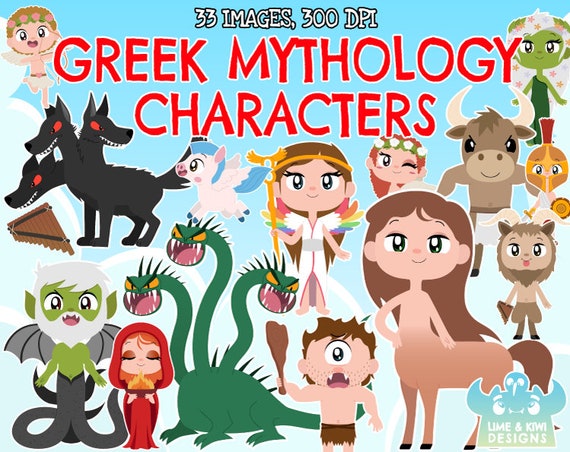This image features the front cover of a children's book, displaying a vibrant and detailed illustration of various Greek mythological characters in cartoon style. The background is a sky blue color, adorned with large white and blue clouds that frame the scene down the left, right, and bottom edges. At the top center, the text "33 images, 300 DPI" is written in small white letters. Directly underneath, the title "Greek Mythology Characters" is prominently displayed in large red letters with a white border.

The cover is brimming with an array of mythological figures. In the upper left corner, a Cupid figure is visible, adding a whimsical touch. Nearby, in the opposite corner, there's a small green creature. Below the title "Greek Mythology," a formidable three-headed black dog with red eyes—likely Cerberus—stands out. To its right, a majestic unicorn adds a touch of magic. Next to the unicorn, a little winged girl holds a goat staff, while adjacent to her, a small elf character appears.

Among other notable figures, a minotaur with large white horns faces the viewer, positioned right of center. Further right at the edge of the image stands a Roman guard. A little goat boy with prominent horns is situated below the guard. In the lower section of the image, a larger female minotaur and a cyclops wielding a billy club take center stage. The cyclops, shirtless and muscular, adds to the menagerie of mythical beings. To the left, a three-headed green dragon bares its teeth menacingly. Next to the dragon, a Little Red Riding Hood figure creates an intriguing anachronism.

In the bottom left corner, a green man with gray hair, a white beard, black wings, and black tentacles emerging from under him completes the fantastic tableau. In the bottom right corner, the label "Lime and Kiwi Designs" gives credit to the designers. The cover, with its lively and eclectic mix of characters, promises an engaging collection of 33 high-resolution images that introduce young readers to the wonders of Greek mythology.